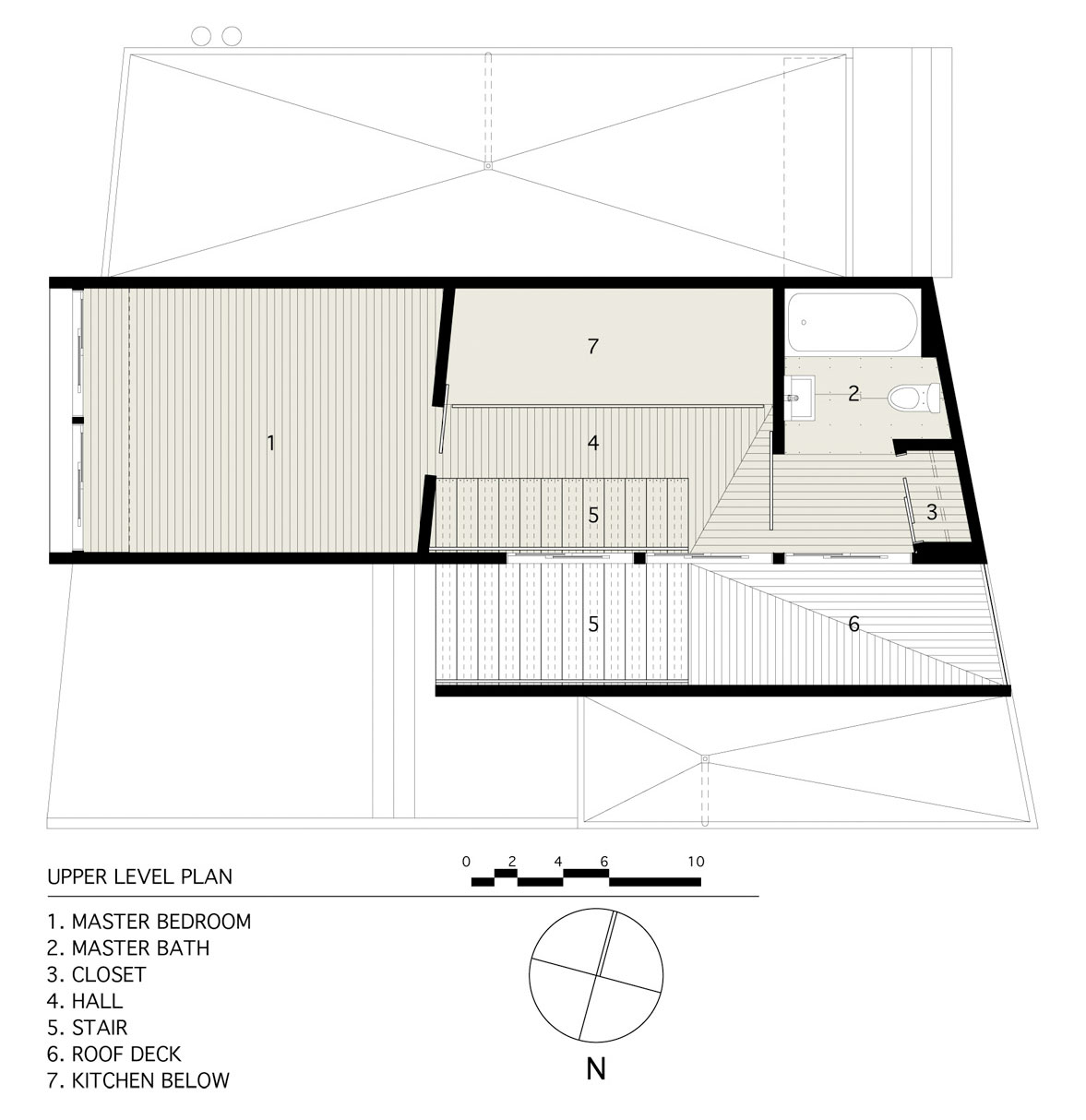The black-and-white image is a detailed architectural drawing, featuring a combination of 2D and 3D perspectives. The plan is titled "Upper-Level Plan" and showcases distinct room layouts and design elements, with various lines of differing thickness. It includes the numbered rooms 1 through 7, each corresponding to a legend located in the lower left-hand corner: 1 - Master Bedroom, 2 - Master Bath, 3 - Closet, 4 - Hall, 5 - Stair, 6 - Roof Deck, 7 - Kitchen Below. The master bath is depicted with fixtures such as a toilet, sink, and bathtub. A compass at the bottom shows the orientation with 'N' for north. Additionally, a scale measurement of 0 to 10 is present, and all the text in the image appears in uppercase.